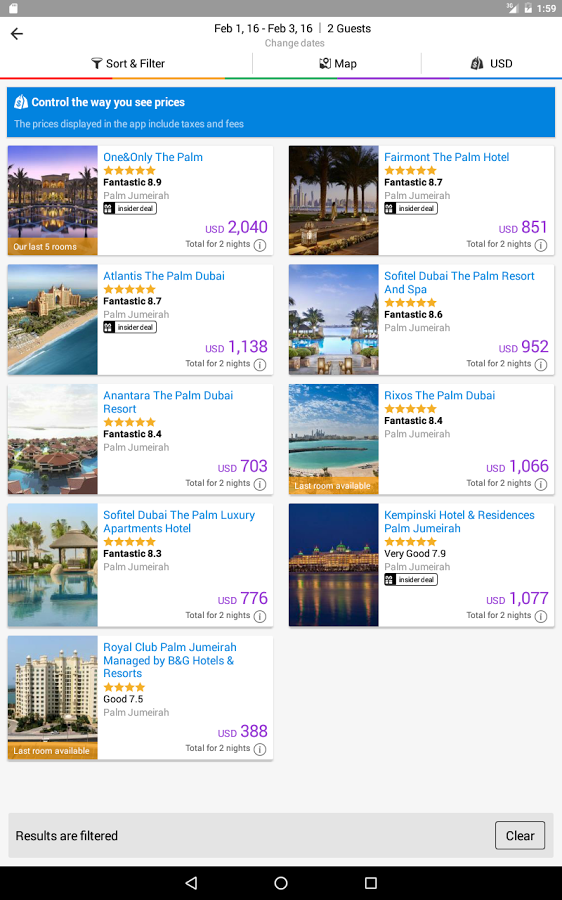The image captures a screenshot from a mobile device displaying the results of a filtered search for hotels. At the bottom left, a gray bar indicates that the results have been filtered. At the top, another gray bar displays a date range, "February 1, 16 to February 3, 16," alongside a slash indicating the search is for "two guests." Below this, a prominent blue bar features a message in white text: "Control the way you see prices." The search results are organized into five rows, with two hotel listings per row, except for the fifth row, which contains only one listing. Each hotel listing includes an image of the hotel and a star rating. All of the hotels listed have a five-star rating, except for the final listing in the bottom left corner, which has a four-star rating.